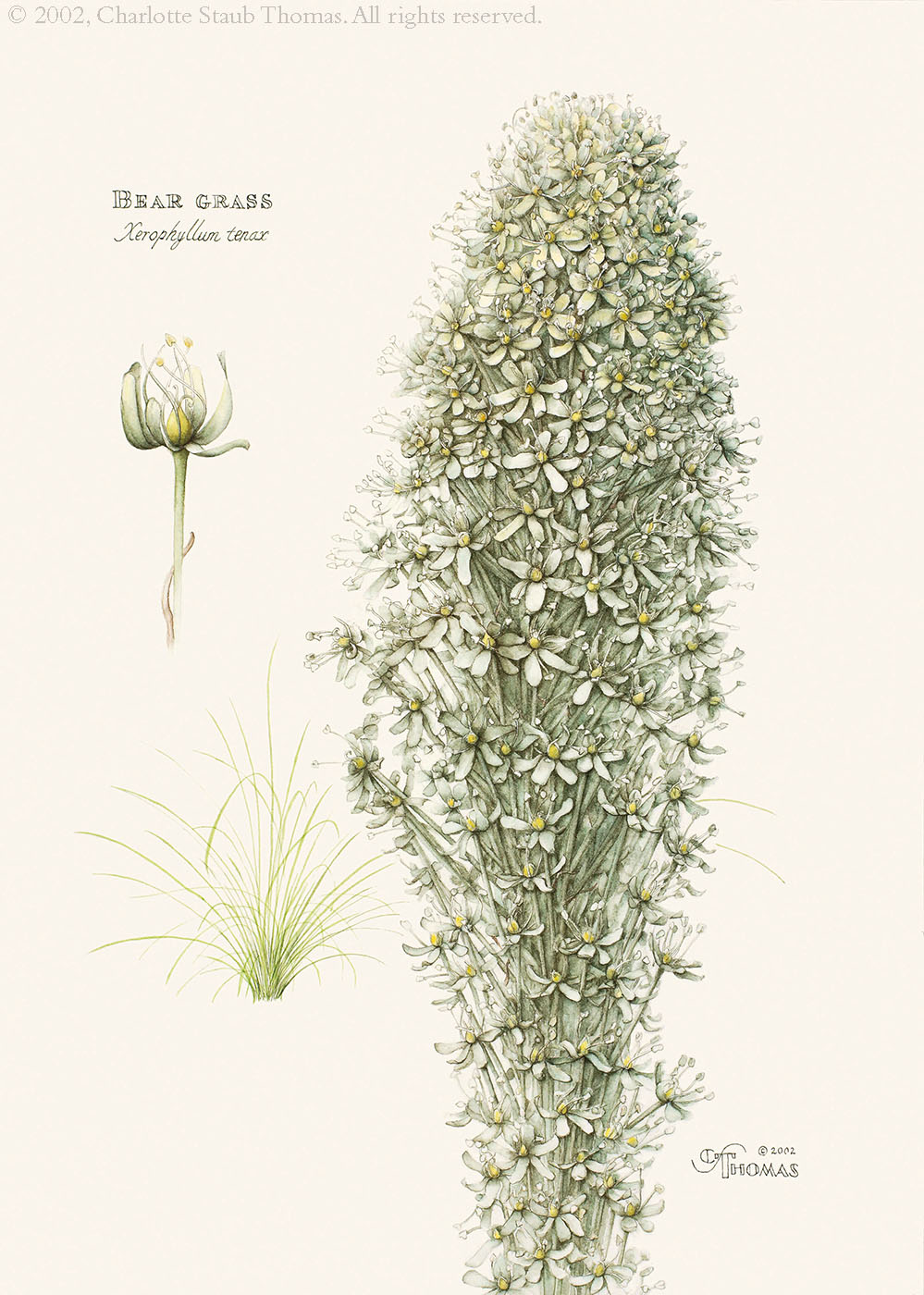The illustration prominently displays a detailed botanical study of Bear Grass (Xerophyllum), created by Charlotte Staub Thomas in 2002, with all rights reserved. The top portion of the image features the artist's copyright in light black lettering, "© 2002, Charlotte Staub Thomas, all rights reserved." Below this, the title "Bear Grass" is presented in bold, darker black text, followed by the scientific name "Xerophyllum" in white text with a black edge.

The right side of the illustration showcases an intricate depiction of Bear Grass flowers, forming a tall bouquet with numerous white blossoms. Each flower is outlined in green tones, providing a sharp contrast against the white background. On the left side, a close-up concept of the Bear Grass is provided, highlighting the yellow bud surrounded by white petals pointing upwards. This detailed segment emphasizes the structure of the plant, showing both the pestle and the slender green leaves below.

Towards the lower right corner, the artist's signature, "CS Thomas, 2002," is visible, reaffirming the artwork's authenticity and creation date. This comprehensive drawing not only celebrates the beauty of Bear Grass but also serves as a scientifically informative piece, enhancing our understanding of the plant's morphology.